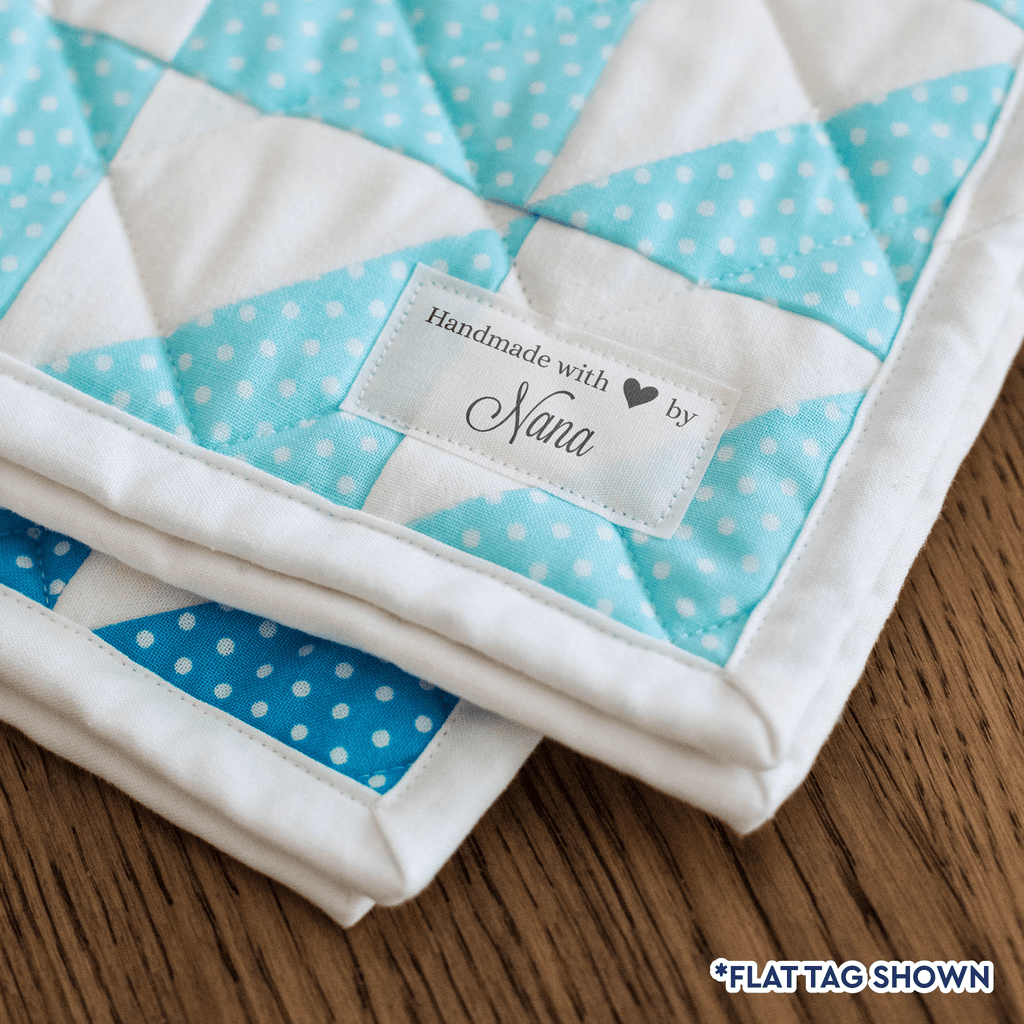This image depicts two handmade baby quilts folded and resting on a hardwood floor. Each quilt is composed of aqua and white patches with white polka dots, arranged in a checkered pattern and crisscrossed with visible stitches. The quilt on top, in a lighter baby blue, features a tag in one corner that reads "Handmade with ❤️ by Nana," with the heart symbol being an emoji. The second quilt underneath shares the same design but uses a deeper blue fabric. Both quilts are trimmed with white fabric along the edges. In the lower right corner of the image, the text "flat tag shown" is displayed in bold dark blue font with a white outline.